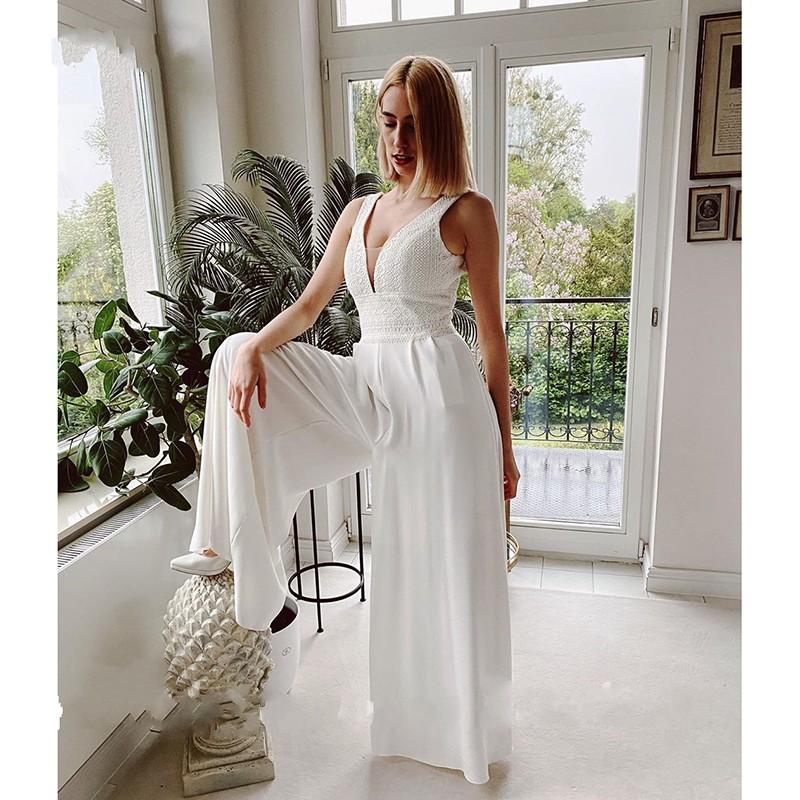In this full-color, professionally taken indoor photograph, a striking young Caucasian blonde woman is the focal point. Positioned centrally within the vertically rectangular frame, she is standing in what appears to be a living room. The room features a window on the far left through which trees can be seen, and a French door that leads to a patio or terrace with a black railing. Outside the door, green leafy bushes and trees are visible, and the sky appears gray yet bright, suggesting a rainy day.

The woman, who has straight blonde hair styled into a bob, is dressed in an elegant, all-white sleeveless pantsuit with a plunging V-neckline and wide-leg pants. She is captured looking downward, posing serenely. Her right leg is propped up on a white statue that resembles a pineapple or an acorn, and she is wearing white shoes. Her right hand rests on her right knee, which is elevated on the statue. A hint of lush green palm trees and possibly other plants can be seen behind her, further enriching the indoor setting with natural elements.